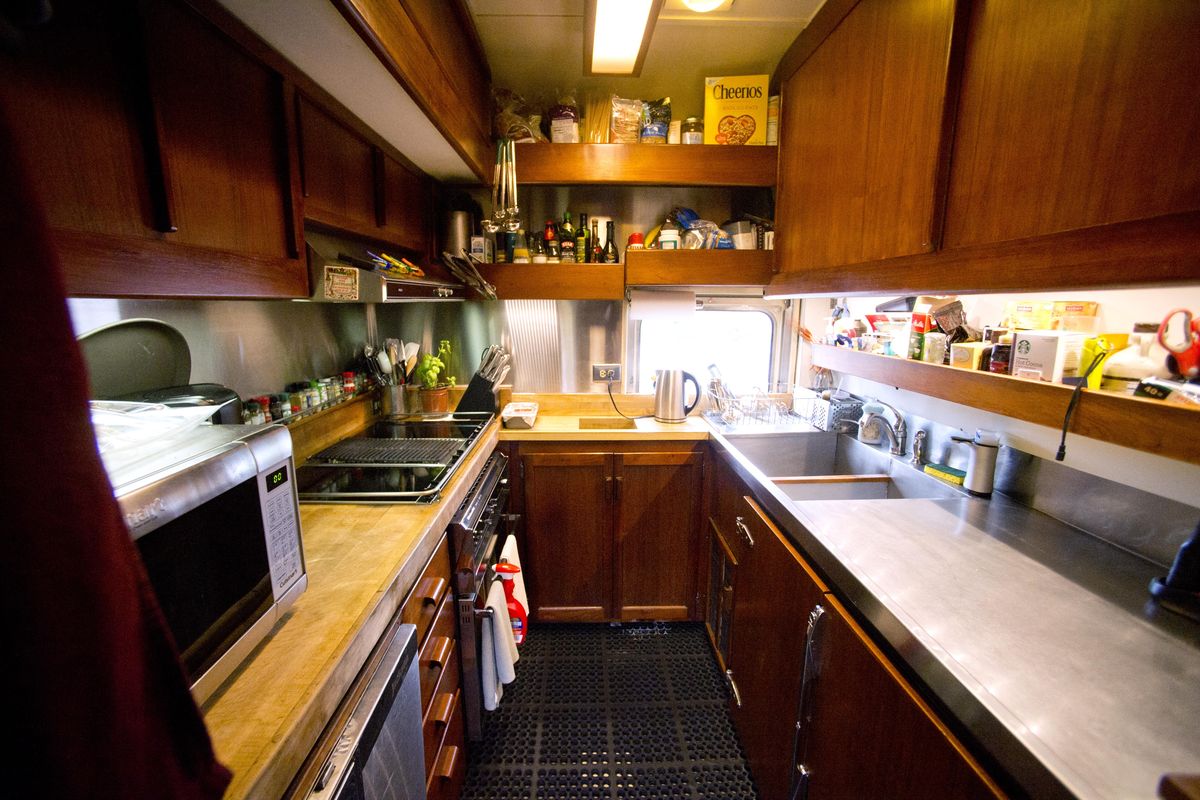The image depicts a narrow, galley-style kitchen, reminiscent of a space you might find in a tiny house, mobile home, or camping trailer. The kitchen features light beige wooden cabinets lining both sides, creating a tight corridor-like space with approximately three feet between them. 

On the left side, towards the rear, there's a small two-burner stovetop positioned above an oven, with a microwave perched on the beige countertop below. Adjacent to the stovetop are hand towels hanging from the oven. The wall above the countertop showcases a few open shelves containing various pantry items, including a box of Cheerios and sauce bottles, likely soy sauce. A green plant or herb is also visible on this side, adding a touch of color.

On the right side, a marble-like countertop spans the length of the kitchen, culminating in a deep double sink. An open shelving unit above the countertop provides additional storage for food items, such as pasta and condiment containers. At the far end of the right counter, there's a silver coffee maker, contributing to the kitchen's functional setup. The floor features a rubber mat with a pattern of holes, ensuring safety and comfort underfoot.